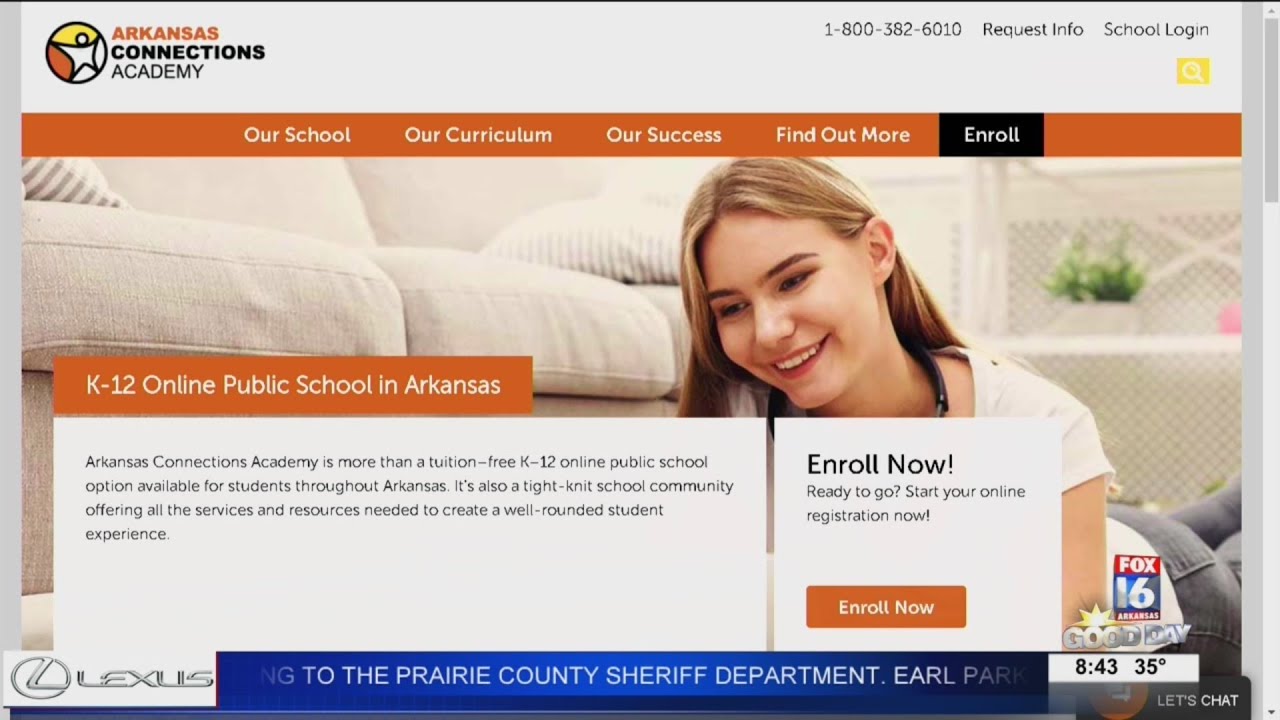This image depicts a screenshot of the Arkansas Connections Academy website. The website features an orange banner at the top with segments labeled "Our School," "Our Curriculum," "Our Success," and "Find Out More." A prominent black button partially overlays the banner with the text "ENROLL" in white, followed by "K-12 Online Public School in Arkansas." Below the banner, a description reads, "Arkansas Connections Academy is more than a tuition-free K-12 online public school option available for students throughout Arkansas. It's also a tight-knit school community offering all the services and resources needed to create a well-rounded student experience." In the background, there is an image of a girl lying on her belly, adding a personal touch to the website.

At the bottom of the screen, a Fox News chyron is visible. On the left side, the Lexus logo is displayed, and on the right, the text "FOX 16 Arkansas" is shown along with the segment title "Good Day." The current time and temperature are also displayed: "8:43" and "35 degrees." The chyron, which has a blue background with white text, features a headline mentioning the Prairie County Sheriff's Department.